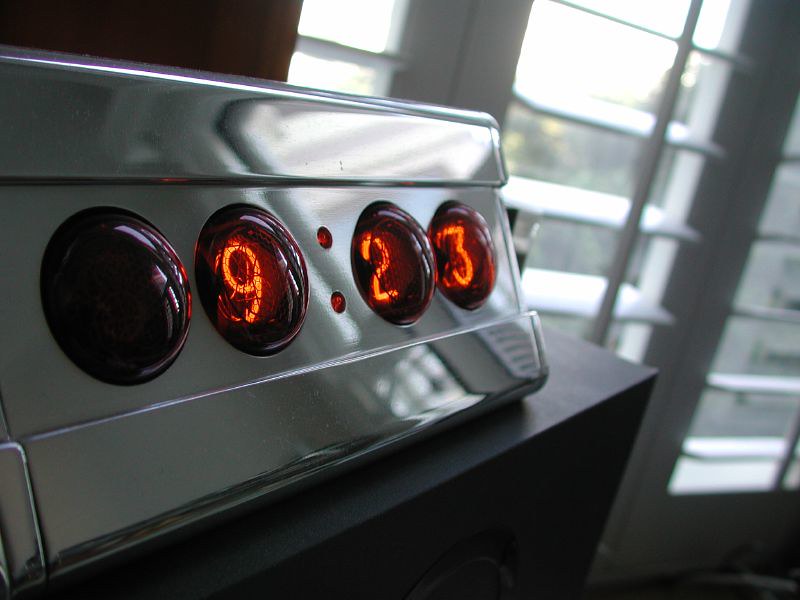This close-up image features a retro-style digital clock crafted from bright stainless steel. The clock's face is distinctive, showcasing four transparent, orange-tinted half-domes made of glass or plastic that display the digital time. The current time shown is 9:23, with the orange backlit numbers clearly visible, separated by a glowing orange semicolon.

The clock's design includes an extruded metal molding at the top and bottom, adding a touch of vintage charm. It rests on the corner of a black table, partially visible in the frame. The background reveals wide-blade white wood shutters on an interior window, fully opened to let in sunlight. Beyond the shutters, blurry green trees bathed in sunlight can be seen, enhancing the nostalgic ambiance of the scene.